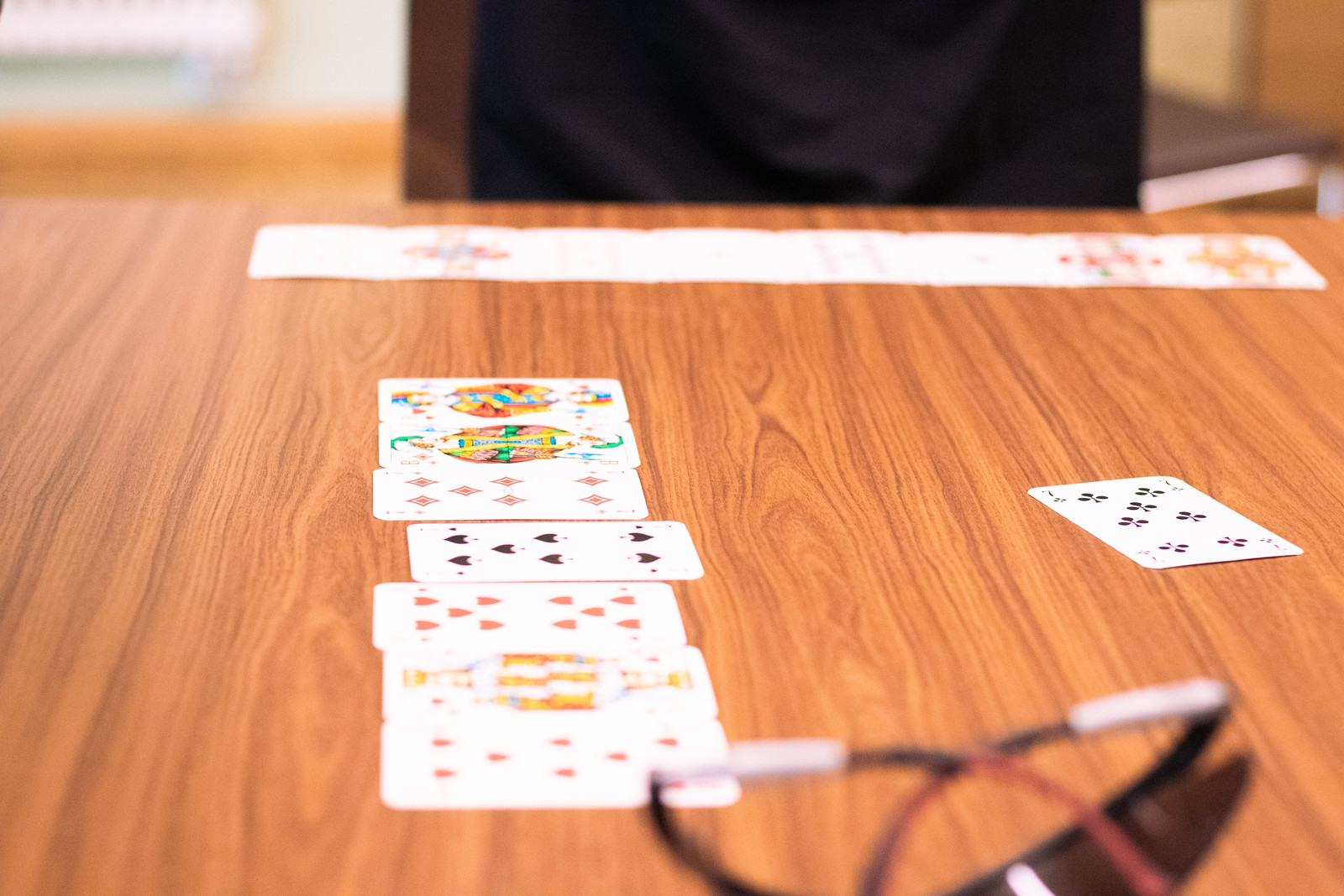This close-up image captures an intricate arrangement of playing cards on a wooden surface. In the distance, partially centered and blending into the background, a black material is discernible, though its specifics remain unclear. 

The playing cards are prominently displayed in two distinct configurations. Furthest from the viewer, a horizontal stack of cards is visible. The topmost card reveals a partial image with a white section leading to another illustration, though the exact details are indistinct due to the overlay of numerous cards.

Closer to the viewer, six cards are meticulously lined up vertically. The sequence begins with a card displaying red hearts, followed by a King card. Next in the sequence is another card adorned with red hearts, succeeded by a card featuring black hearts. After this, a card with red diamonds appears, and the line-up concludes with two Joker cards placed side by side.

Beneath this arrangement, a seven of clubs is oriented lengthwise towards the viewer, adding depth to the spread. Adjacent to the playing cards, a pair of narrow-looking sunglasses lies face down, with the earpieces folded over one another. These sunglasses are slightly blurred, softening the overall crispness of the scene. 

The image, rich with detail, presents a snapshot not just of playing cards, but of a moment intricately composed on a humble wooden surface.